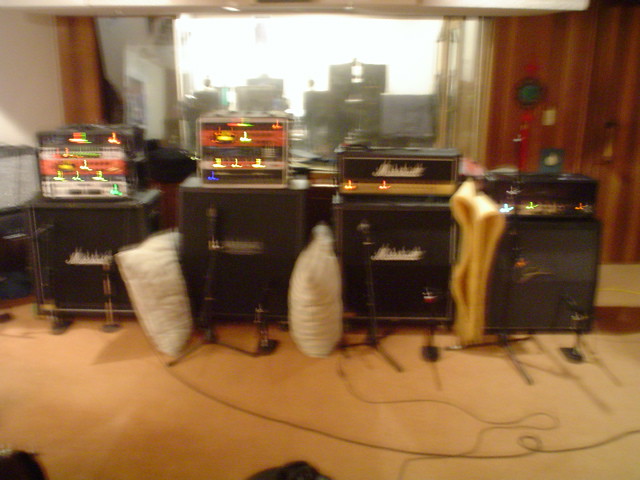The photograph is a somewhat blurry image of a recording studio setup. It prominently features various pieces of music equipment arranged on their respective cases. In the center, there are square-shaped modules such as soundboards, mixers, and amplifiers, with visible control panels featuring colorful buttons in blue, green, yellow, and red. Some of these modules bear white text that reads "Marshall." To the front of these modules lie microphones on the ground, amidst white pillows and foam padding for sound insulation. The ground is light brown and scattered with black cable cords. In addition, tripods with mounted mics can be seen turned at different angles. Another notable detail includes the presence of brown cabinets to the right side of the image, supporting rectangular boxes that rest on top of the musical equipment. The scene is bathed in a blur, suggesting low camera quality or motion at the time of capture, making fine details somewhat difficult to discern. Overall, the arrangement and colors indicate a bustling, albeit slightly chaotic, recording environment.